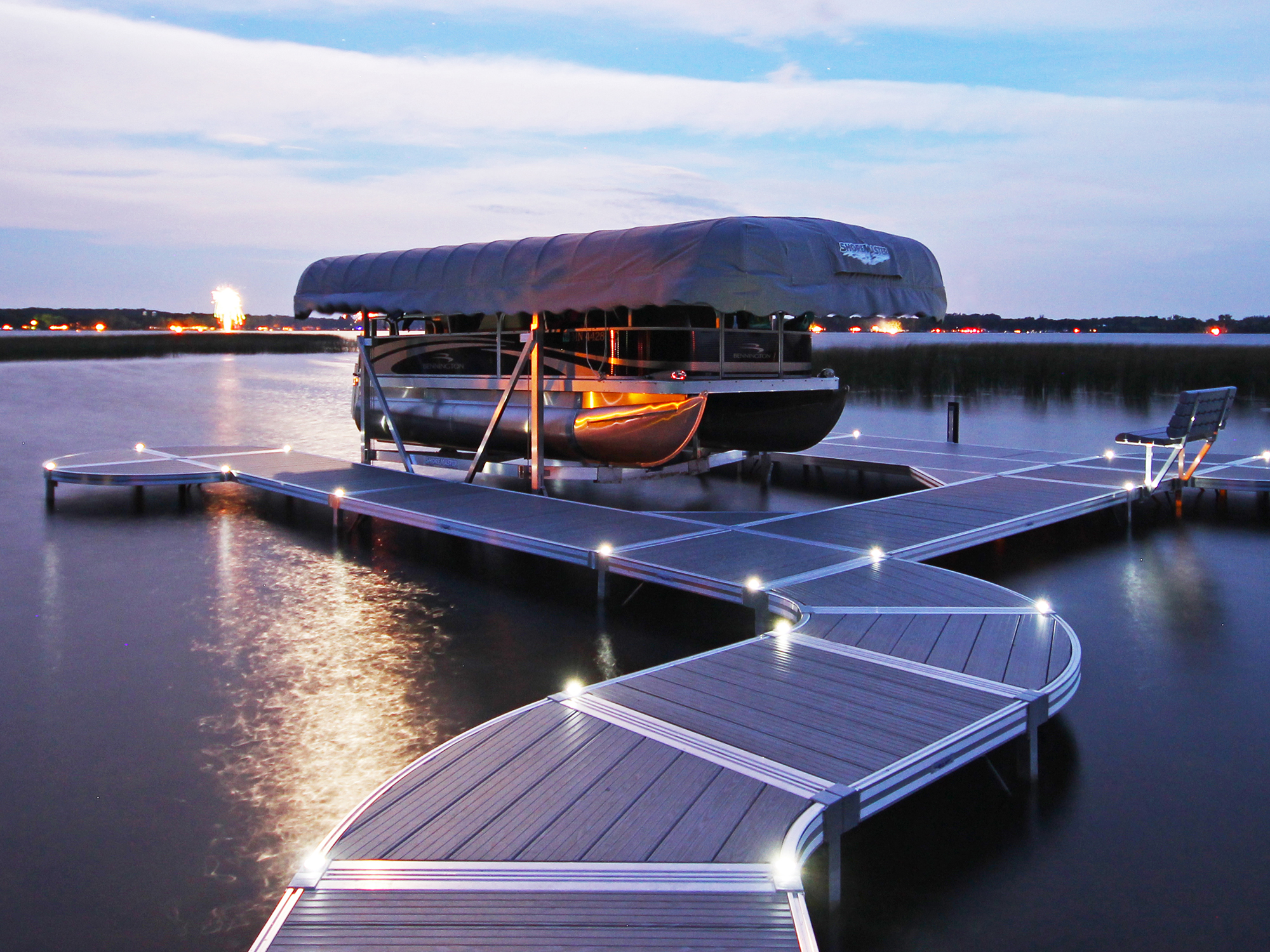In the photograph, a serene scene unfolds with docks extending into the calm sea, which is a dark blue hue reflecting shimmering white light from above. The docks, made of grey wood, have light bulbs attached along their edges, emitting a soft, white glow. In the middle of the docks, a black boat with a large rectangular blue canopy is parked, its precise shape adding an intriguing element to the composition. The water is flat and calm, mirroring the tranquil setting. In the distance, the further shore is faintly visible under the blue sky adorned with scattered white clouds, encapsulating a moment of peaceful beauty.